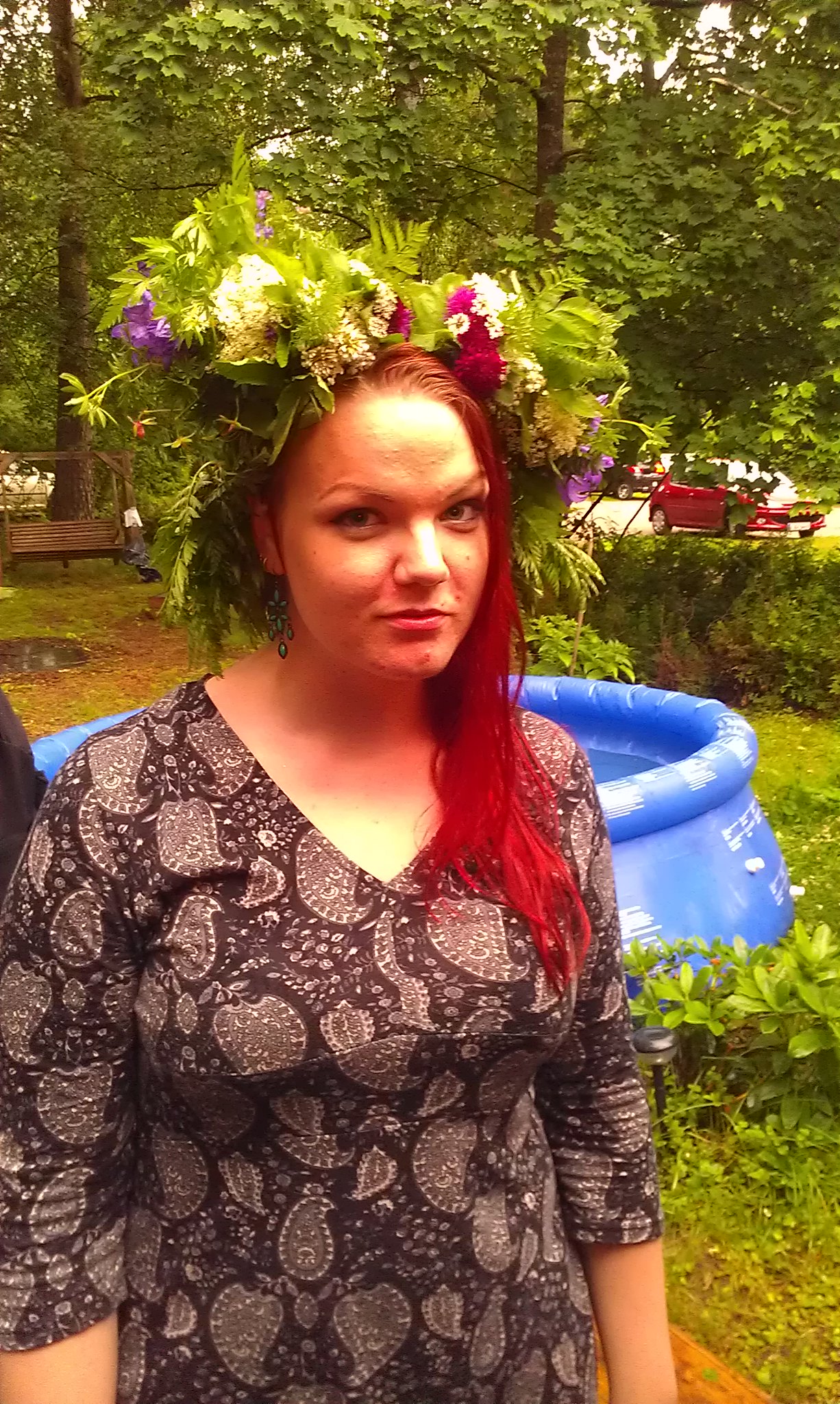The photograph captures a woman with long, vibrant red hair adorned with an intricate flower crown featuring various blooms, including pink, white, and purple flowers, interspersed with lush green leaves. She is wearing a paisley-patterned top in shades of black, gray, and brown. The woman, likely in her late 20s or early 30s, stands slightly to the left but is mostly centered in the frame, looking directly at the camera with a slight grin on her face. In the background, there's an above-ground blue pool, a wooden swing, and a scenic backdrop of trees and shrubs. To the far right, a red car and a black SUV are visible. The setting appears to be a pleasant daytime outdoor scene, with a bright sky enhancing the overall tranquility of the image.